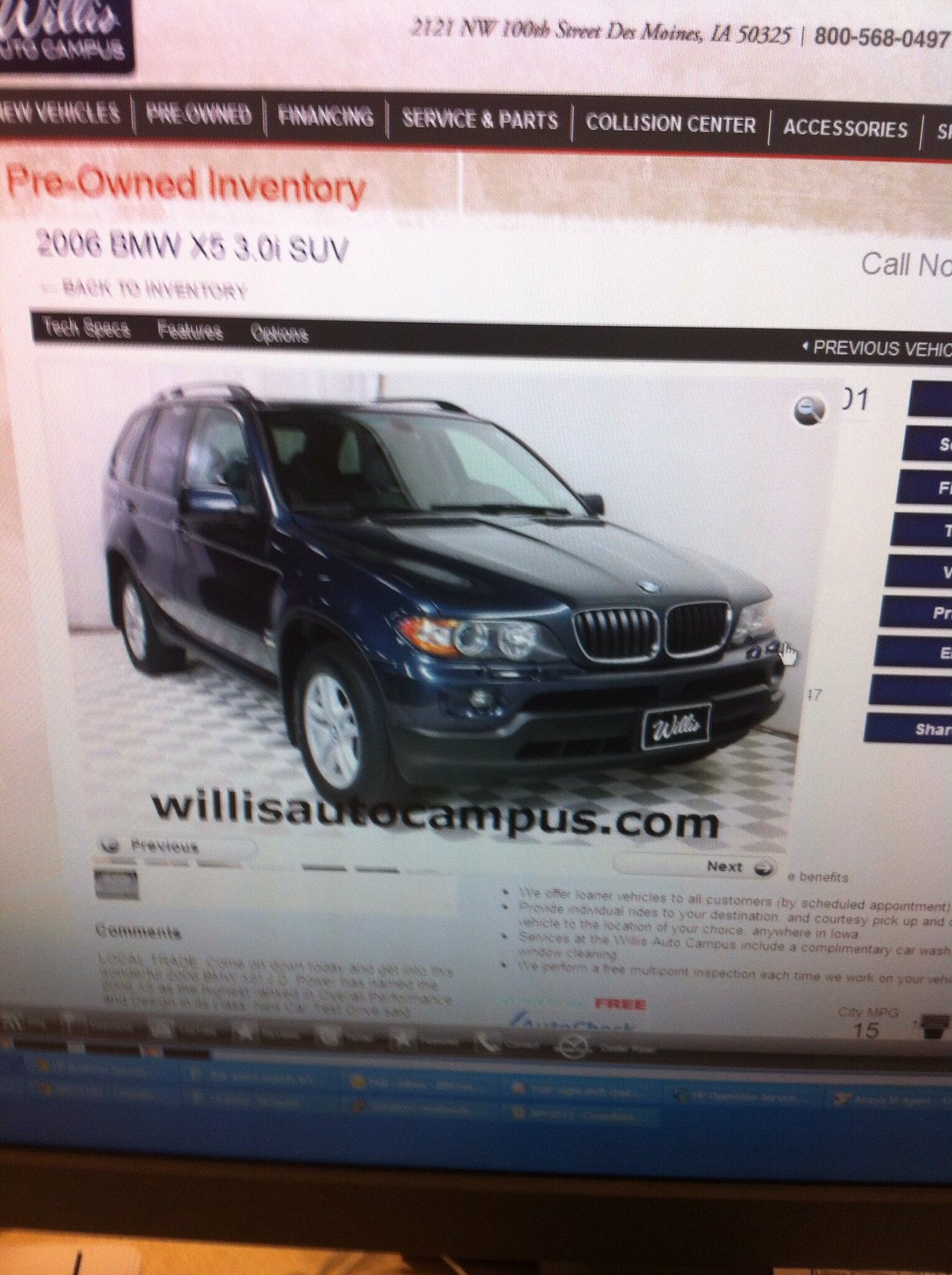The image depicts a photograph taken with a cell phone of a computer screen displaying a car sale advertisement on a dealership website. The webpage features the pre-owned inventory section, highlighting a 2006 BMW X5 3.0i SUV in a bright blue color. The car is shown in a showroom, looking shiny and free of scratches. The website, identified as willysautocampus.com, includes various categories along the top, such as new vehicles, pre-owned, financing, service and parts, collision center, and accessories. The advertisement includes a clear picture of the vehicle and options for sharing and viewing more details on the right side. The car's license plate reads "Willys," the name of the selling company.